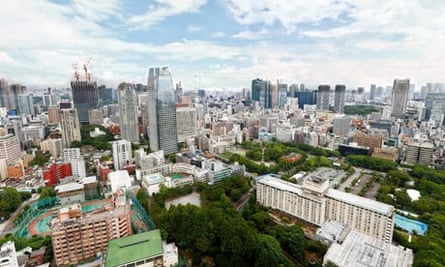This detailed aerial view of a metropolitan area captures an expansive urban landscape framed by a sky that's predominantly cloudy with patches of blue. In the lower right corner of the horizontal, rectangular image is a prominent large white building, likely a multi-story hotel or motel, with what appears to be a rooftop swimming pool. Adjacent to this building is a sign, possibly indicating the establishment's name. Towards the left side of the image, a red multi-story building stands tall, fronted by a green billboard. Between these two structures lies a verdant area brimming with bright, vibrant green trees, suggesting a park or recreational space. In the background, an extensive sea of skyscrapers and various smaller buildings creates a dense cityscape, giving the impression of unbroken urban sprawl. The lower left-hand corner hints at a stadium or car garage, accompanied by a fenced sports area, adding to the mix of urban elements. The sky above is dotted with interspersed white clouds, adding a dynamic overhead contrast to the bustling city below.